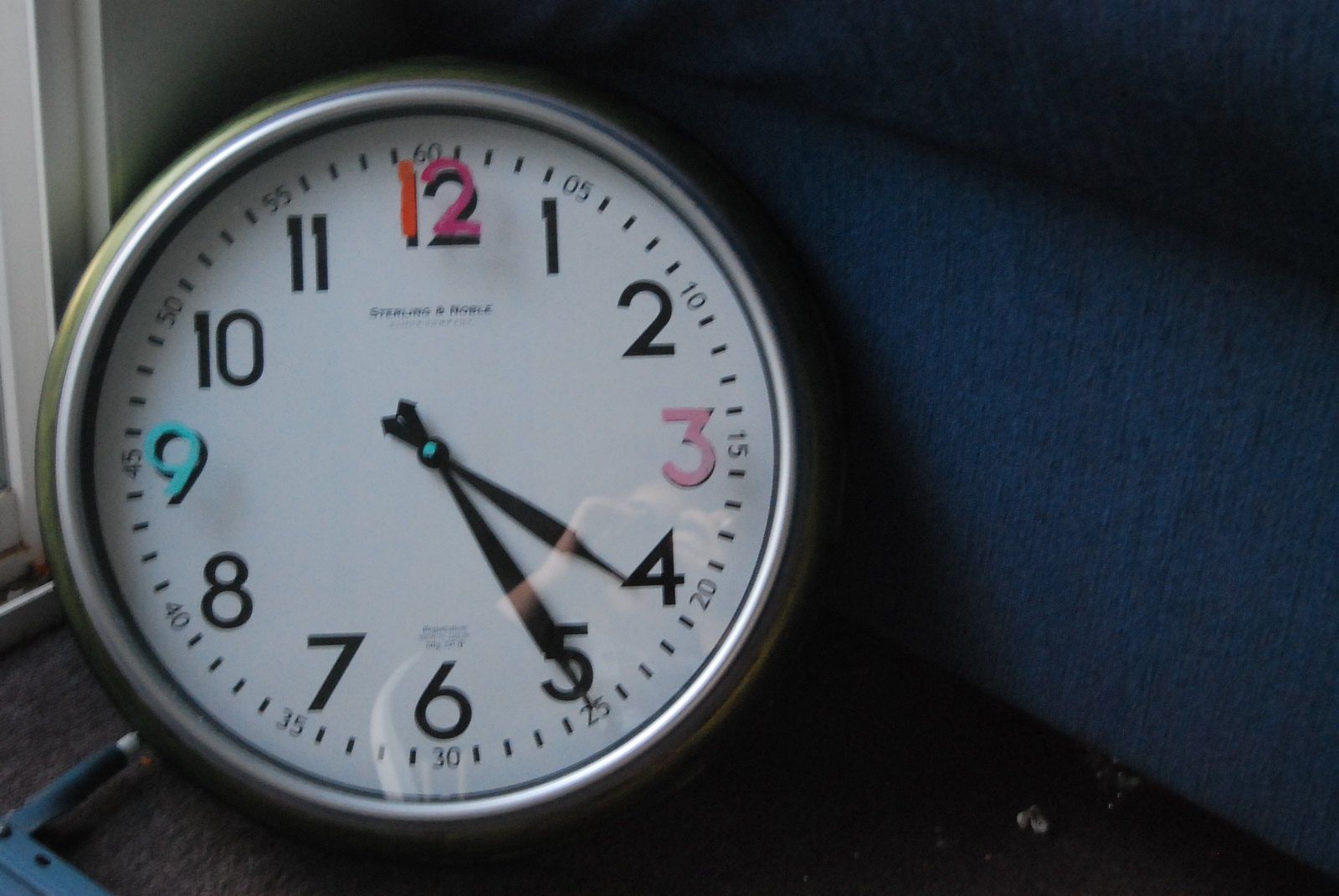In the image, a round clock with a silver frame leans against the intersection of two walls. The wall to the right appears to be a dark shade of blue, casting deep shadows around the clock, contributing to the dimly lit ambiance of the scene. The other wall seems white and features an opening that might be a window, adding subtle contrast to the composition.

The clock face displays numbers 1 through 12, with the numerals 1 and 2 in red and pink respectively. The number 3 also stands out in pink, while the number 9 is in a light blue color. The remaining numbers are black. The clock includes minute markings, with every 5-minute interval labeled sequentially from 0 to 60, located where the number 12 typically is.

Both the minute and hour hands are black, indicating the time as approximately 4:25. This detailed portrayal captures not only the appearance but also the specific features and setting of the clock.